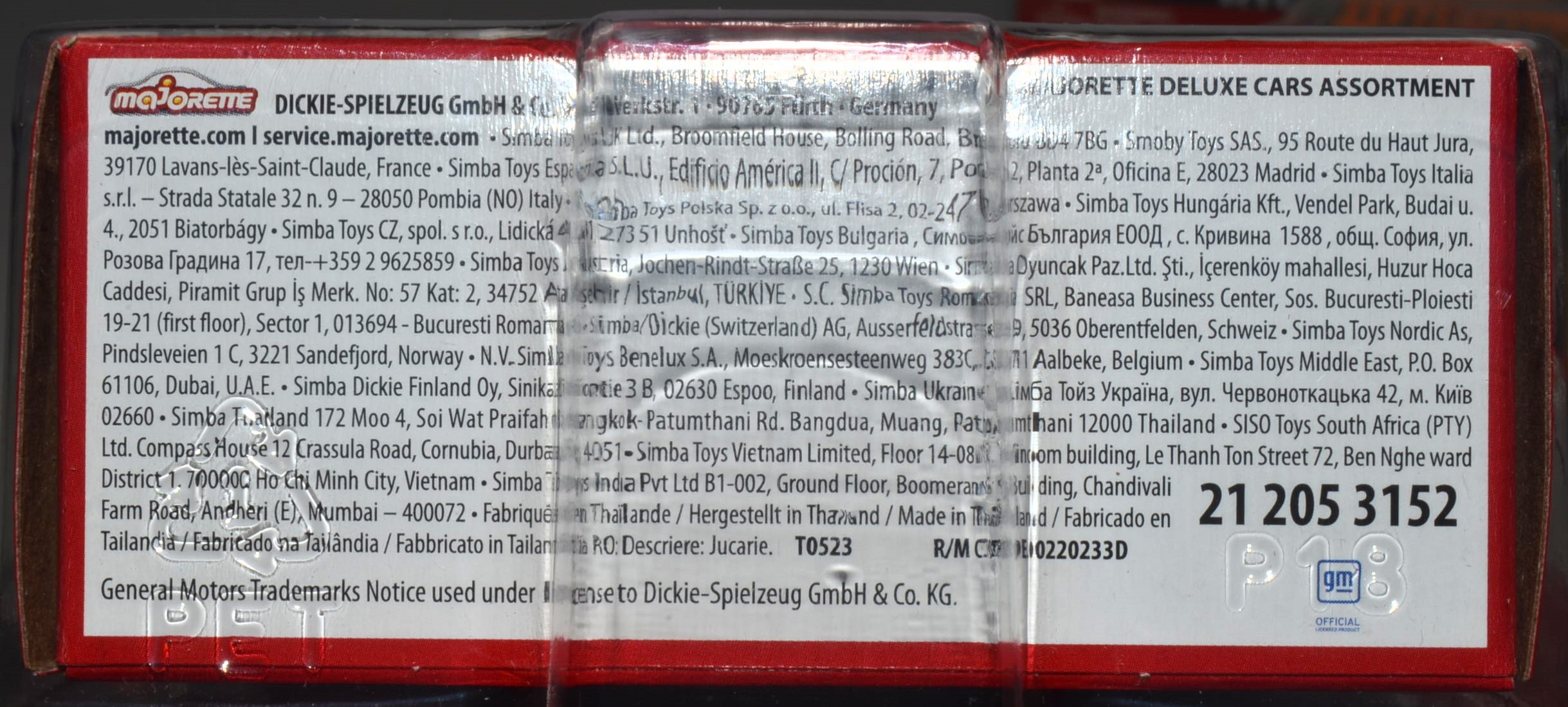A detailed close-up image showcases the side of a red cardboard package, with both ends securely closed. The side panel, encased in a clear plastic wrapping that reflects light and creates a noticeable glare, features a white background. Bold black lettering on this white side spells out "Majorette Deluxe Cars Assortment," indicating the contents of the box. The overall packaging suggests a well-protected, high-quality toy car selection.